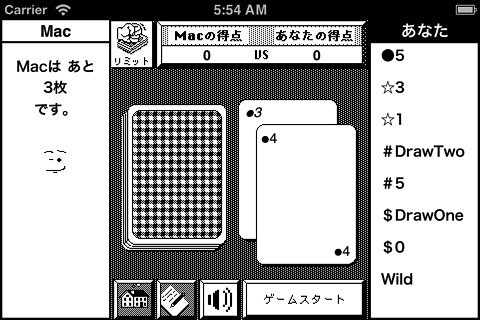The image captures a black and white screenshot of an online digital card game on either a phone or computer screen. At the top of the screen, user interface elements are visible, including a Wi-Fi signal icon, the word "carrier," the time displayed as 5:54 AM, and a battery icon. The screen also features the word "Mac" along with text in an Asian language, possibly Chinese or Japanese. In the center of the screen, there's a game in progress with a stack of cards face down sporting a houndstooth plaid design. Beside the stack, two face-up cards show numbers "3" and "4," marked with black dots instead of traditional card suits. To the right, a tally column lists various game elements: numbers "5," "3," and "1" each labeled with stars, "draw two" marked with a pound sign, another "5" with a pound sign, "draw one" with a dollar sign, "zero" with a dollar sign, and an entry labeled "wild." The top part also depicts an image of a fist hitting the cards with the text "Mac, zero, US," and more Asian language characters.